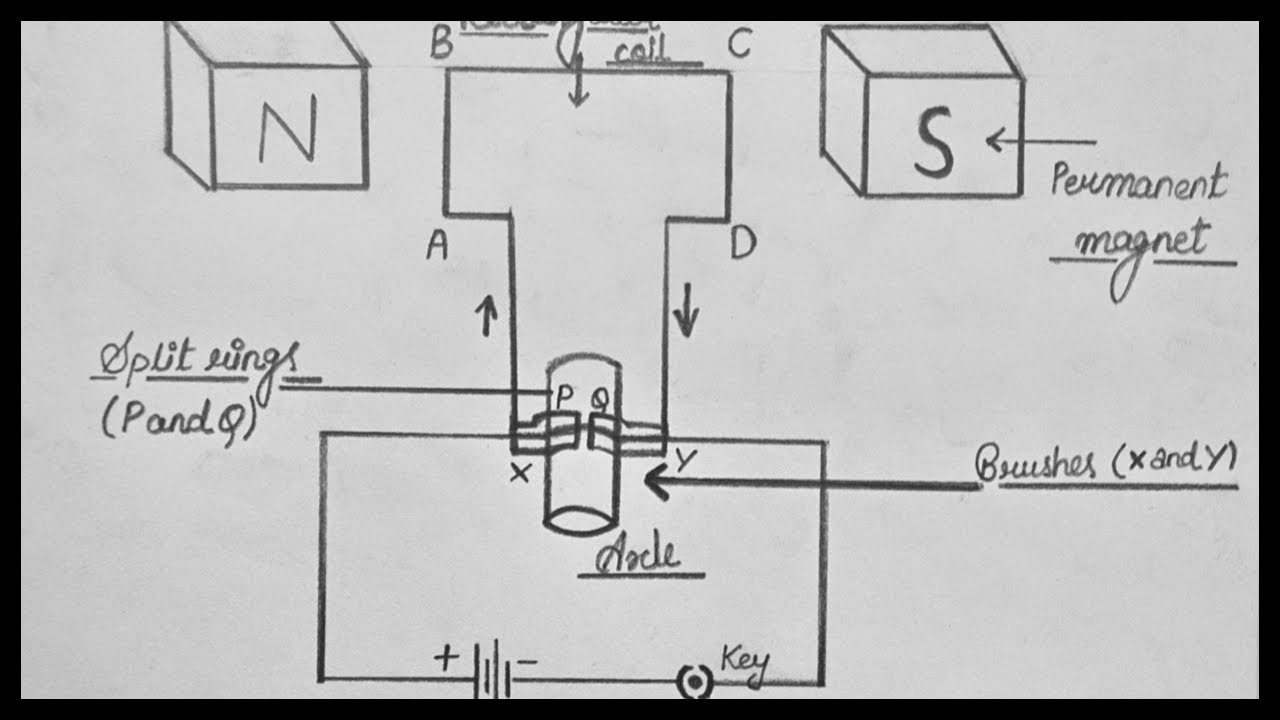The image is a detailed hand-drawn pencil diagram on off-white paper, framed by a black outline, depicting a mechanical or electrical design. On the upper left, there is a 3D cube labeled "N" and on the upper right, another 3D cube labeled "S" with an arrow pointing to it, along with the handwritten note "permanent magnet." Central to the drawing is a T-shaped structure with labeled corners: B at the upper left, C at the upper right, A at the lower left, and D at the lower right. There are arrows indicating motion; one points up below A, and another points down below D. Below the top of the T is a cylindrical shape, around which labels identify "split rings P and Q" and "brushes X and Y." Beneath the cylinder is a large rectangle with a "plus" and "minus" sign, the words "a coal" and "key" written next to it, and additional annotations. This intricate blueprint suggests a complex mechanical or electrical system.